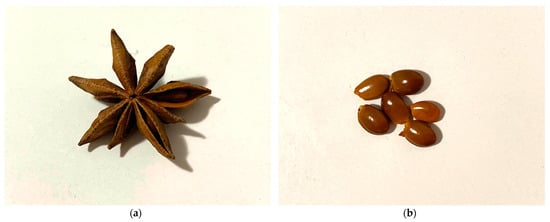Displayed are two separate images, each on its own piece of light cream to slightly bluish cloth. The image on the left features a star anise, viewed from above, resembling a brown, star-shaped flower with seven distinct pods radiating from the center. The background on this image has a light pinkish hue, possibly influenced by the lighting, and a notable shadow is cast from the star anise towards the bottom right. Below this star anise, there is a lowercase black "a" enclosed in parentheses.

The image on the right shows six shiny, brown oval objects that mirror the star anise in color. These objects, likely beans or nuts, also lie on a light pinkish background cloth and cast shadows to the bottom right, similar to the star anise. Below these six items is a lowercase black "b" in parentheses. Both images emphasize a shared reflective quality of the items depicted and a somewhat uniform background.